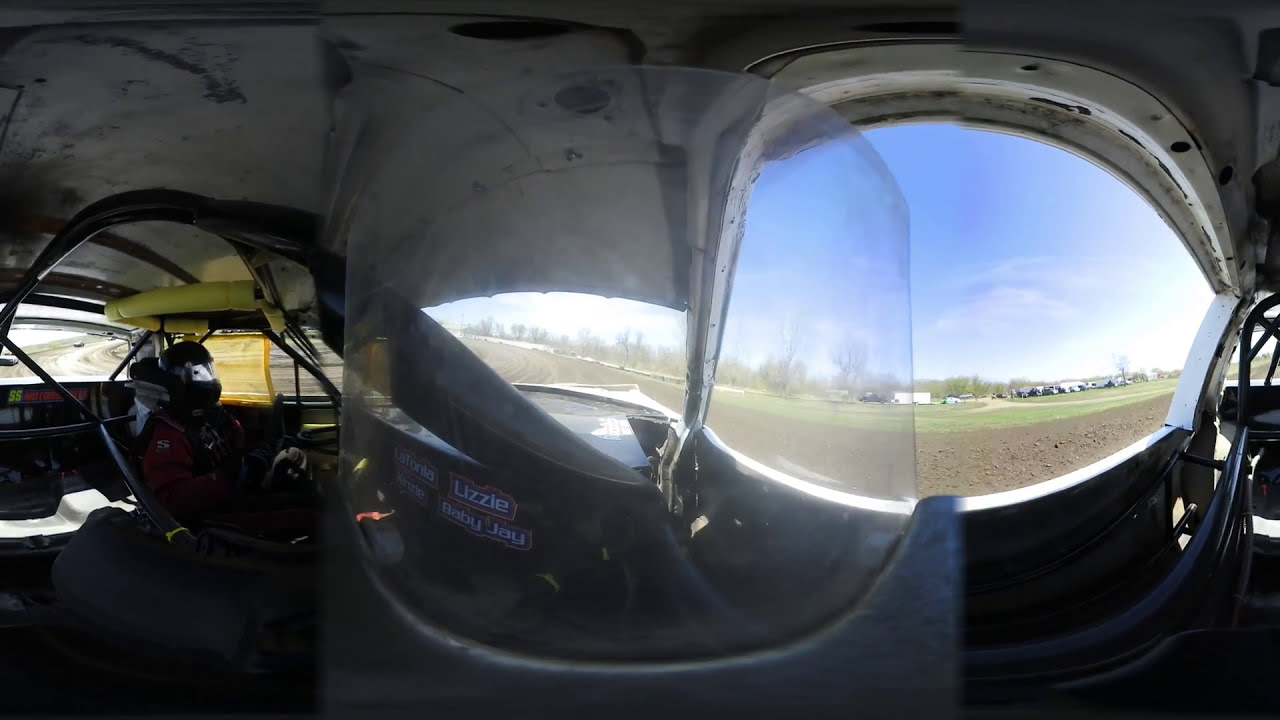The photograph captures the interior of what appears to be a race car, evident from its sparse, industrial design and the presence of a roll cage. The interior is devoid of typical car features such as windows or liners, with a metal roof and a dark, somewhat gritty atmosphere. On the left side of the image, a driver can be seen seated, clad in a red suit and black helmet, their identity obscured. Yellow foam padding is visible on the roll cage surrounding the driver, emphasizing safety measures. Positioned centrally in the image is a glass or perspex screen mounted in a grey holder, and some text can be discerned, reading "Lizzie" and "Baby Jay" in white. The vantage point likely suggests the photograph was taken from the passenger seat. Looking out through a somewhat arched window without glass, the exterior shows a bright blue sky with a few clouds, a dirt track with patches of green grass, and trucks parked off in the distance. Further beyond, trees line the horizon, contributing to the scene's vivid outdoor setting.